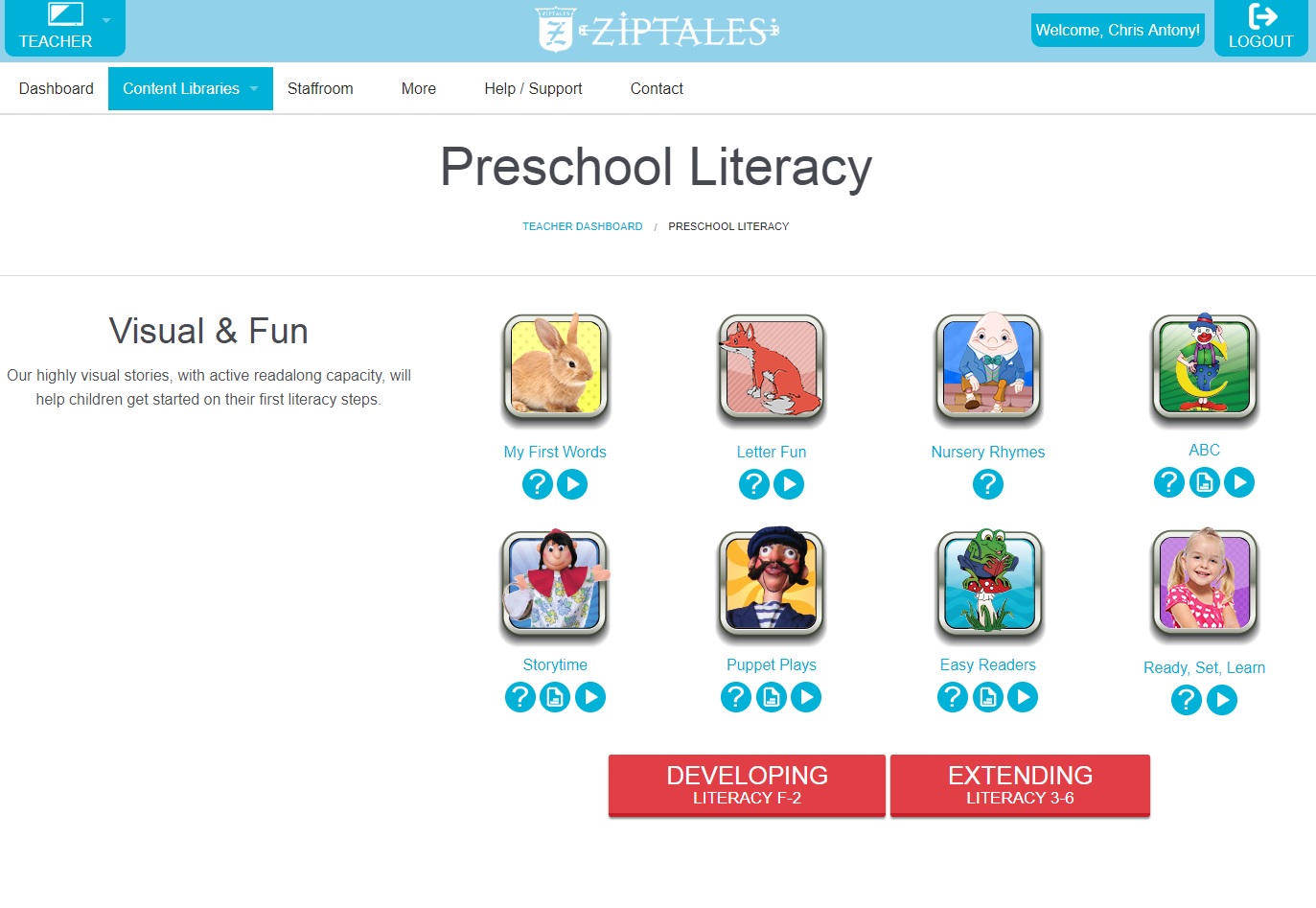This horizontal image, likely from a website accessible via computer or smart device, showcases a user interface designed for educational purposes. The top section features a light blue rectangular banner. In the upper left corner, within a darker blue box, there is a clickable text labeled "Teacher." The upper right corner similarly displays a darker blue box with "Welcome Chrissy, Anthony," and a "Logout" button.

Centered near the top of the image, there is a white "Ziptales" logo with a small icon immediately to the left. Below the logo, a navigation menu spans horizontally, presenting several options in black font, except for the currently selected option, "Content Libraries," which is highlighted in blue. Other menu items include "Dashboard," "Staff Room," "More," "Help," "Support," and "Contact."

The central part of the image prominently displays "Preschool Literacy" in bold black text. Directly beneath, "Teacher Dashboard" appears in blue, followed by "Preschool Literacy" in black.

On the left side of the image, the text "Visual and Fun" is emphasized in black, indicating that "Our highly visual stories with active read-along capacity will help children get started on their first literacy steps."

Visually engaging icons are arranged in two rows of four, each depicting either a person or an animal, including an image of a bunny labeled "My First Words." These clickable icons are interspersed with symbols such as a question mark and a triangle, representing different interactive options.

The lower section of the image differentiates educational levels with "Developing Literacy F to 2" and "Extending Literacy 3 to 6," both highlighted in red, guiding users to appropriate literacy content for various age groups.